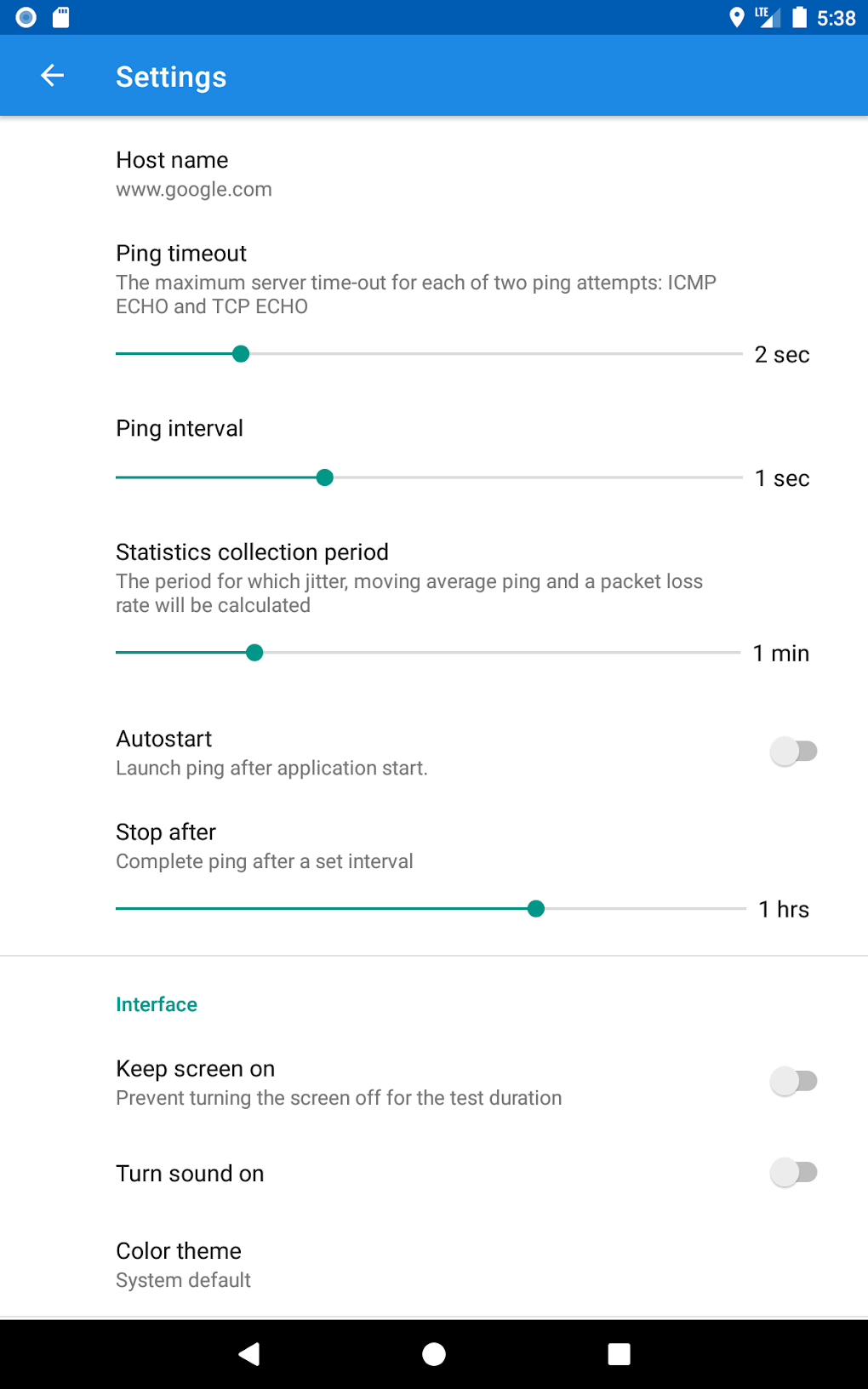Screenshot of a website interface with detailed ping settings:

At the top of the image, there is a darker blue banner featuring a round white circle, followed by a white SIM card icon. On the right side of the banner, the location icon, battery status, the time displayed as 5:38, and a cell signal indicator reading "LTE" in capital letters are visible. Below the banner, a lighter blue background contains a left-pointing arrow and the word "Settings" in white print with a capital "S."

The primary content begins with "Host Name: www.google.com," followed by a section for "Ping Timeout," which specifies, "The maximum server timeout for each of two ping attempts, ICMP echo, and TCP echo." This section includes a slider line with a green circle set to "2 seconds." 

Next is the "Ping Interval" section, also featuring a slider line with a green circle set to "1 second." 

Following this, the "Statistics Collection Period" section details, "The period for which jitter moving average ping and packet loss rate will be calculated," with a slider showing "1 minute." 

The "Auto Start" section, describing "Launch ping after application start," is not selected.

Finally, there is a "Stop After" section stating, "Complete ping after a set interval," which is chosen and set to "1 hour." 

Additional interface options shown are "Keep Screen On" and "Turn On Color Theme."